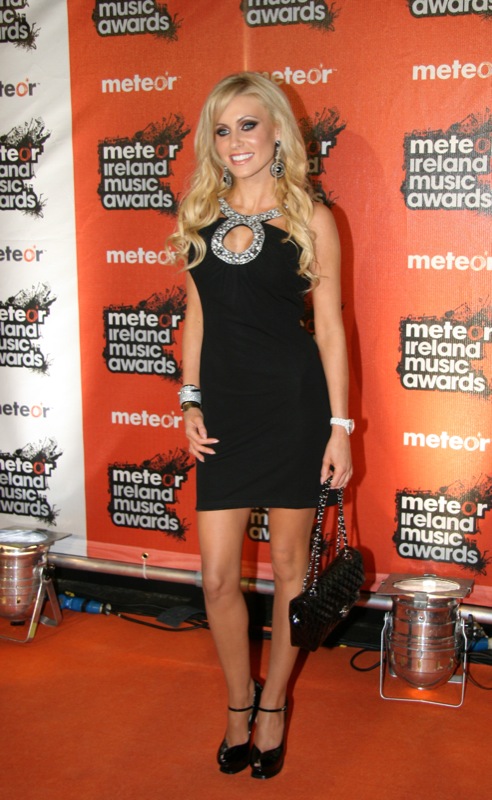In this professionally lit, glamorous photograph taken at the Meteor Ireland Music Awards, a stunning celebrity poses on an orange carpet reminiscent of the iconic red carpet events. The blonde woman, with her long, curly hair styled into side-swept bangs, showcases her elegance in a little black dress adorned with rhinestone trim and a keyhole opening at the chest. Her ensemble is further elevated with a rhinestone bracelet, large dangly earrings, and a chic black handbag. Complementing her attire, she wears black high heels and a white watch on her wrist. Her makeup is impeccably done, enhancing her bright blue eyes and lovely smile. The background features an orange and white backdrop with the Meteor Ireland Music Awards logo repeated in a pattern, emphasizing the event's branding as she poses gracefully, angled slightly to the left. The overall scene is perfectly captured, showcasing the celebrity's poised and stylish appearance amidst an atmosphere of high-profile glamour.